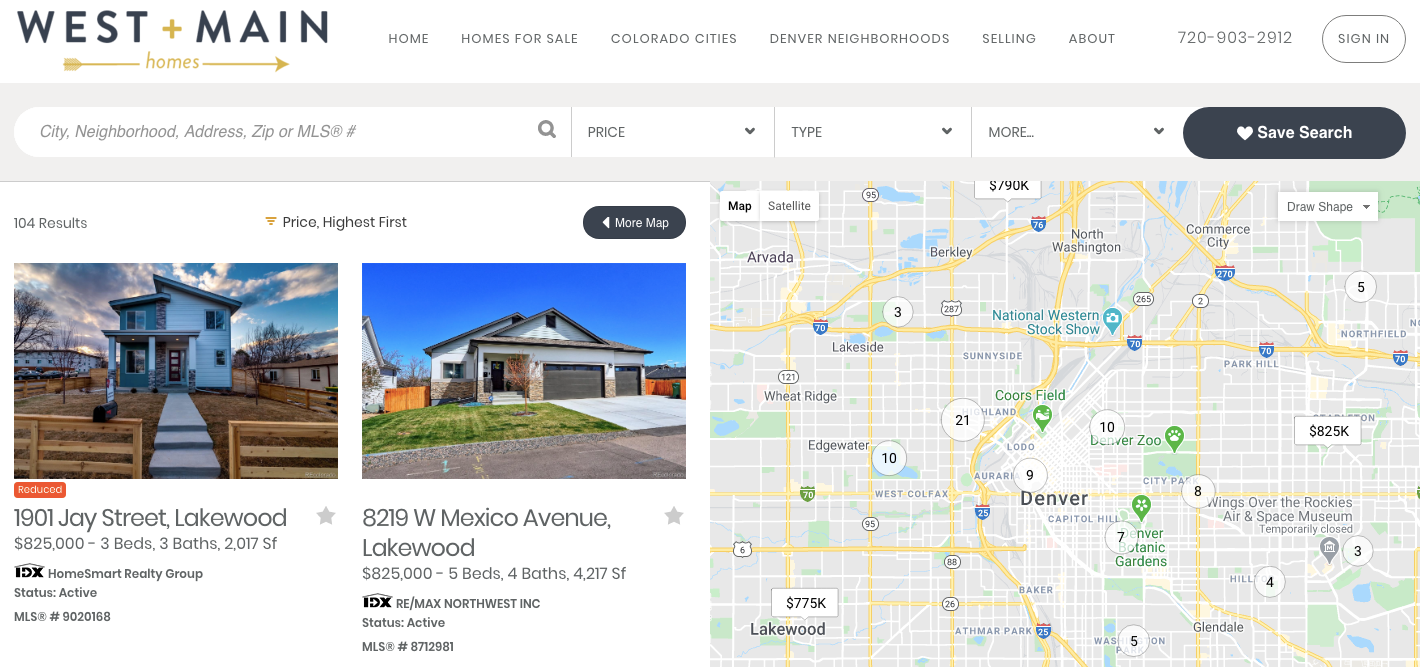The image displays a real estate website named "West Main Homes," highlighting available homes for sale. On the left, two specific properties are showcased. The first property, situated at 1901 Jay Street in Lakewood, is listed at $825,000 and features three bedrooms, three bathrooms, and covers 2,017 square feet. Adjacent to it is another listing at 8219 W Mexico Avenue, also in Lakewood, priced similarly at $825,000. However, this home boasts five bedrooms, four bathrooms, and an expansive 4,217 square feet.

On the right side of the image, there's a map illustrating various property locations and their respective price ranges in different zones. For example, the average home price in Lakewood is noted to be $775,000, while areas east of Denver exhibit higher prices, averaging around $825,000, with further variations observed in northern regions.

The website offers more than just listings; it enables users to explore homes for sale across different Colorado cities and Denver neighborhoods, provides a platform to sell their own homes, and includes a login feature for personalized access.